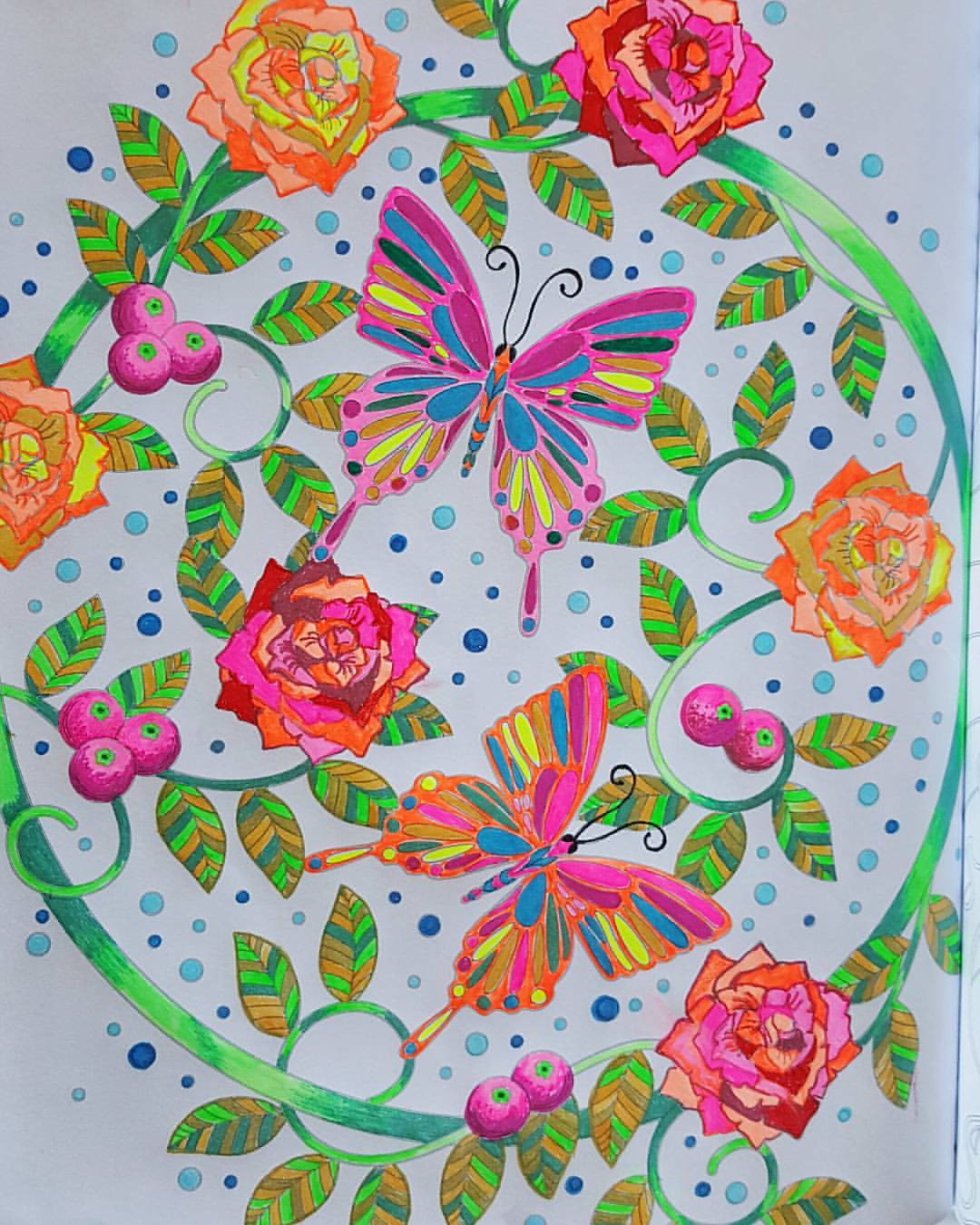A beautifully executed drawing, captured in a photograph that, while bright and in focus, unfortunately cuts off parts of the artwork. The drawing itself is rendered in high-quality markers of various colors, showcasing a verdant green ring from which lush plants, flowers, and berries sprout. The focal point of the drawing is a pair of butterflies, their wings adorned with a striking palette of pink, purple, and red hues. The rich green tones of the leaves and vines provide a vibrant contrast, bringing the entire scene to life.